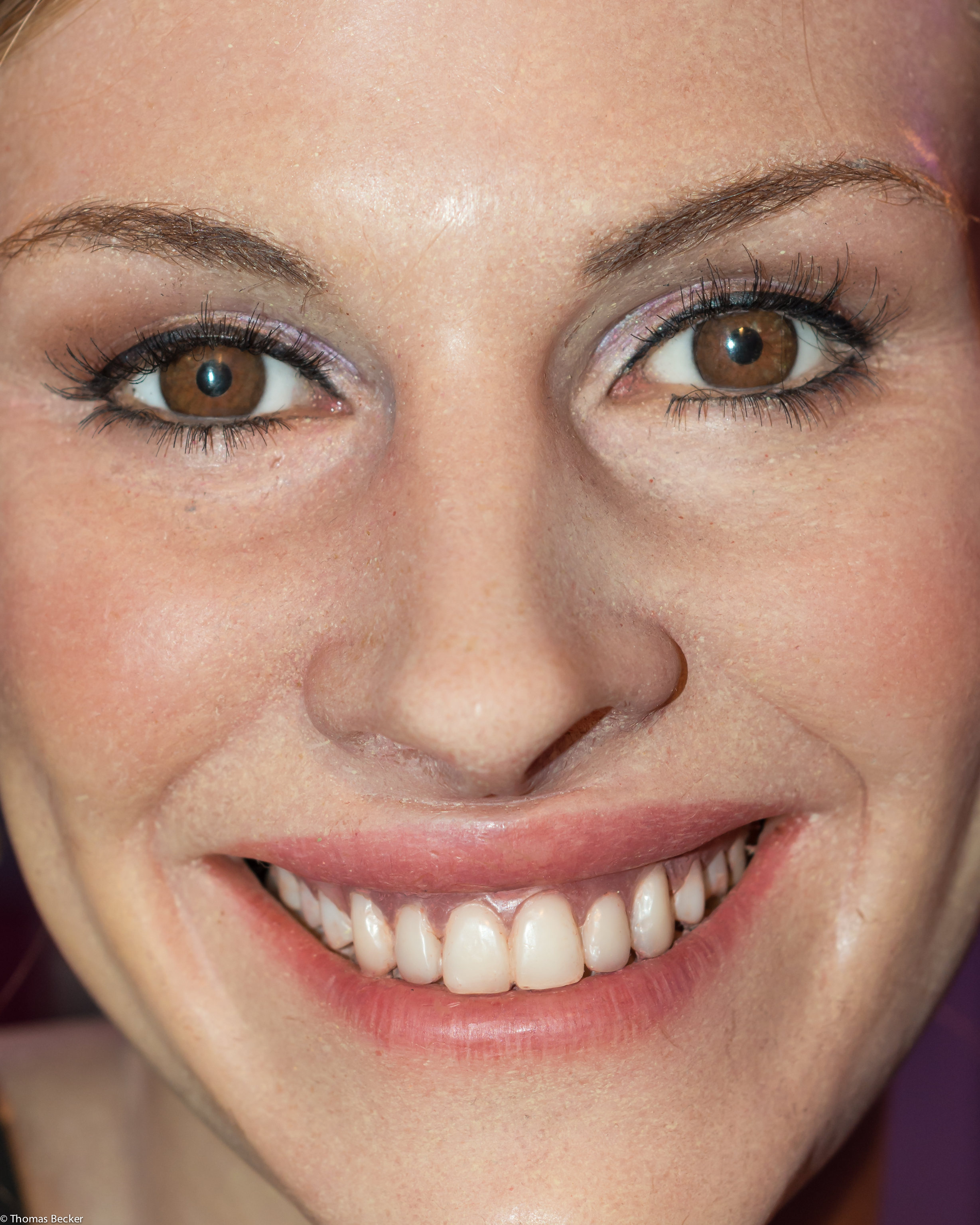This vibrant, close-up photograph features a smiling white woman centrally positioned against a maroon background. Her face, occupying the entire frame, reveals detailed features: she has brown eyes accentuated by black eyeliner and even, brown eyebrows. Her cheeks have a slight brown and red tint, and she's wearing light pink lip gloss on her narrow lips. The woman's healthy smile showcases her top teeth and brown-tinged gums. Part of her right shoulder is visible, adding to the intimate framing of this image.